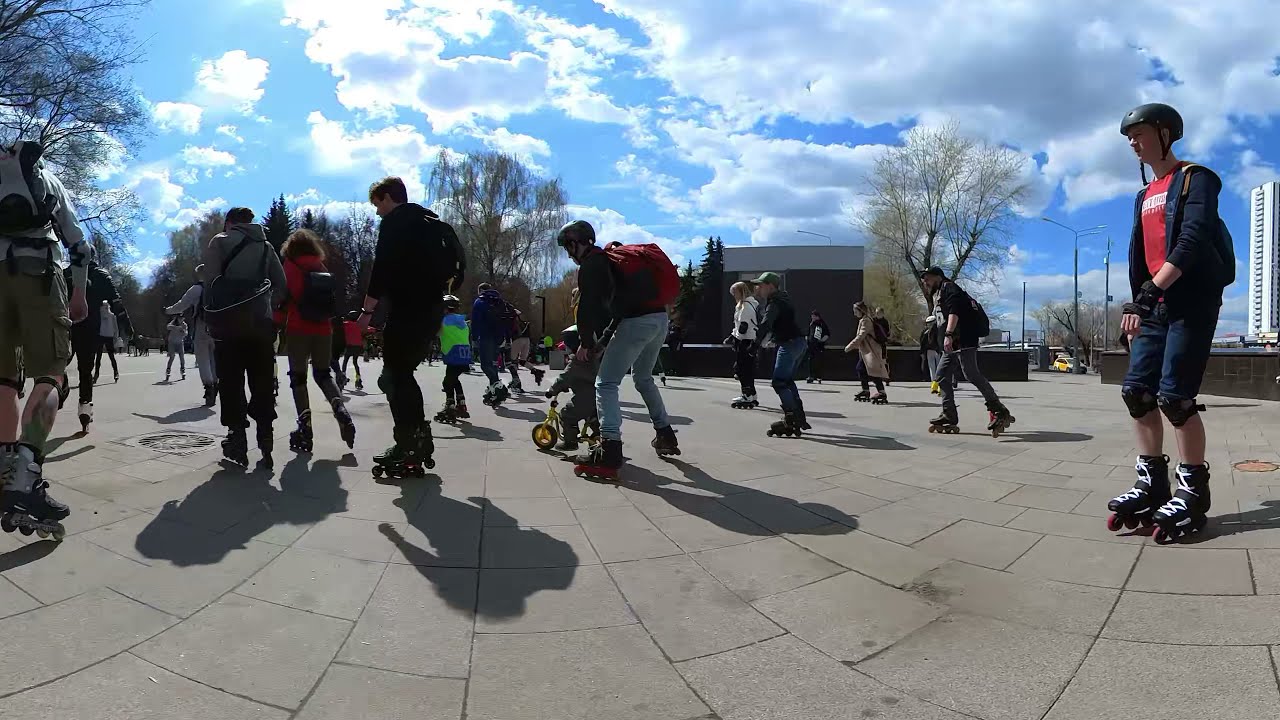The photograph captures an energetic outdoor scene set in a city park during the fall, evidenced by the fallen leaves and the crisp, partly cloudy sky with blue, white, and grayish clouds. The ground is clearly visible and comprised of cement squares and rectangles. Approximately 100 people, including men, women, and children, are participating in what appears to be a family-friendly rollerblading marathon, interspersed with some skateboarding activities. 

Central to the image, a man with a red backpack and helmet assists a young child on a tricycle. To the right, another man in a red shirt, short blue pants, and a black helmet stands on rollerblades, looking to the left. The background features a low-standing building which could be a concession stand, along with a taller building and trees showcasing their seasonal transition. The scene is bustling with activity, showcasing a vibrant community enjoying a day of outdoor sports and family bonding.